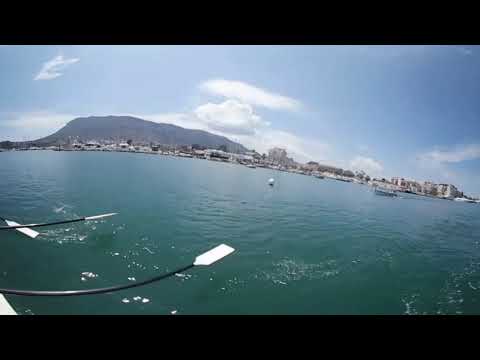This image depicts a serene ocean view from the vantage point of a paddleboat, evidenced by the black oars with white tips dipping into the dark greenish-blue water in the lower left corner. The expansive body of water stretches out towards the horizon, meeting a shoreline that curves gently upward from the right to the left of the frame. The shoreline features a range of buildings dotted along the landmass, with a towering black mountain situated in the distance. The sky above is a clear blue with a scattering of clouds. Towards the right side of the image, there are smaller boats on the water and a distinct white buoy floating prominently. The varied colors present include deep blues, greens, blacks, whites, grays, and tans, capturing the essence of an outdoor, mid-day ocean scene.